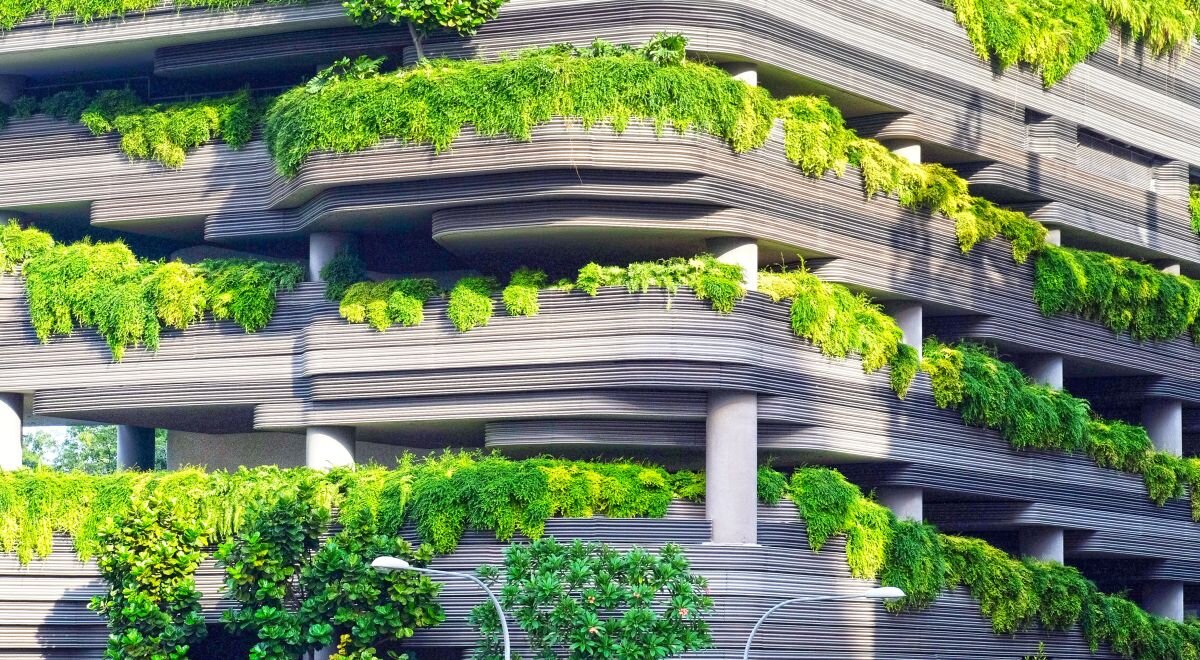This image showcases the corner and facade of a massive, multi-story building designed with sleek, modern architecture. The structure features several levels stacked upon each other, with prominent pillars visible both inside and outside, contributing to its grand and intricate appearance. The exterior has a smooth texture, predominantly in shades of gray and black, interspersed with horizontal lines running from right to left. Adding a touch of nature, lush green and yellow bushes and grass emerge from the edges of the floors, creating a stark contrast against the building's monochromatic palette. At the base of the building, streetlight poles are visible, with the tops of two lamps facing opposite directions—one towards the left and the other towards the right—adding to the urban environment depicted in the scene.